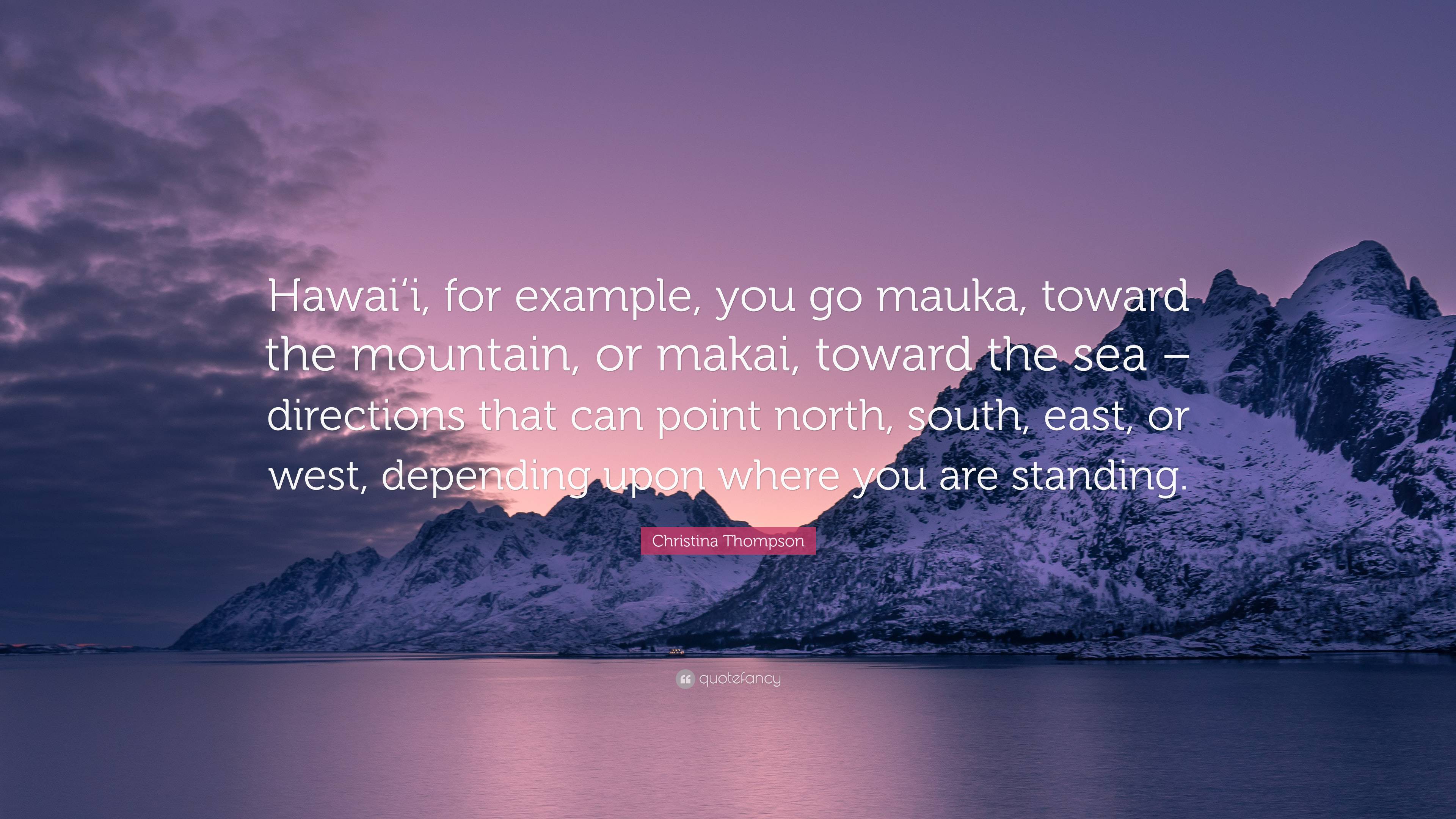The image features a striking, serene landscape at either sunset or sunrise, characterized by a vivid, gradient sky transitioning from deep purple to light pink and purple hues near the horizon. Below the glowing sky, jagged, snow-covered cliffs or a craggy mountainous island stretch horizontally across three quarters of the image, starting from the lower left and extending to the right. The scene appears calm, with the reflection of the pink and purple sky shimmering on the calm body of water in the foreground. Sparse clouds linger on the left side of the otherwise clear sky. At the center of the image, a quote in white text reads: "Hawaii, for example. You go Mauka, toward the mountain, or Makai, toward the sea, directions that can point north, south, east, or west, depending upon where you are standing," attributed to Christina Thompson. Below the quote, the text "Quote Fancy" is subtly displayed. The overall composition evokes tranquility and introspection, enhanced by the harmonious blend of natural elements and thoughtful words.